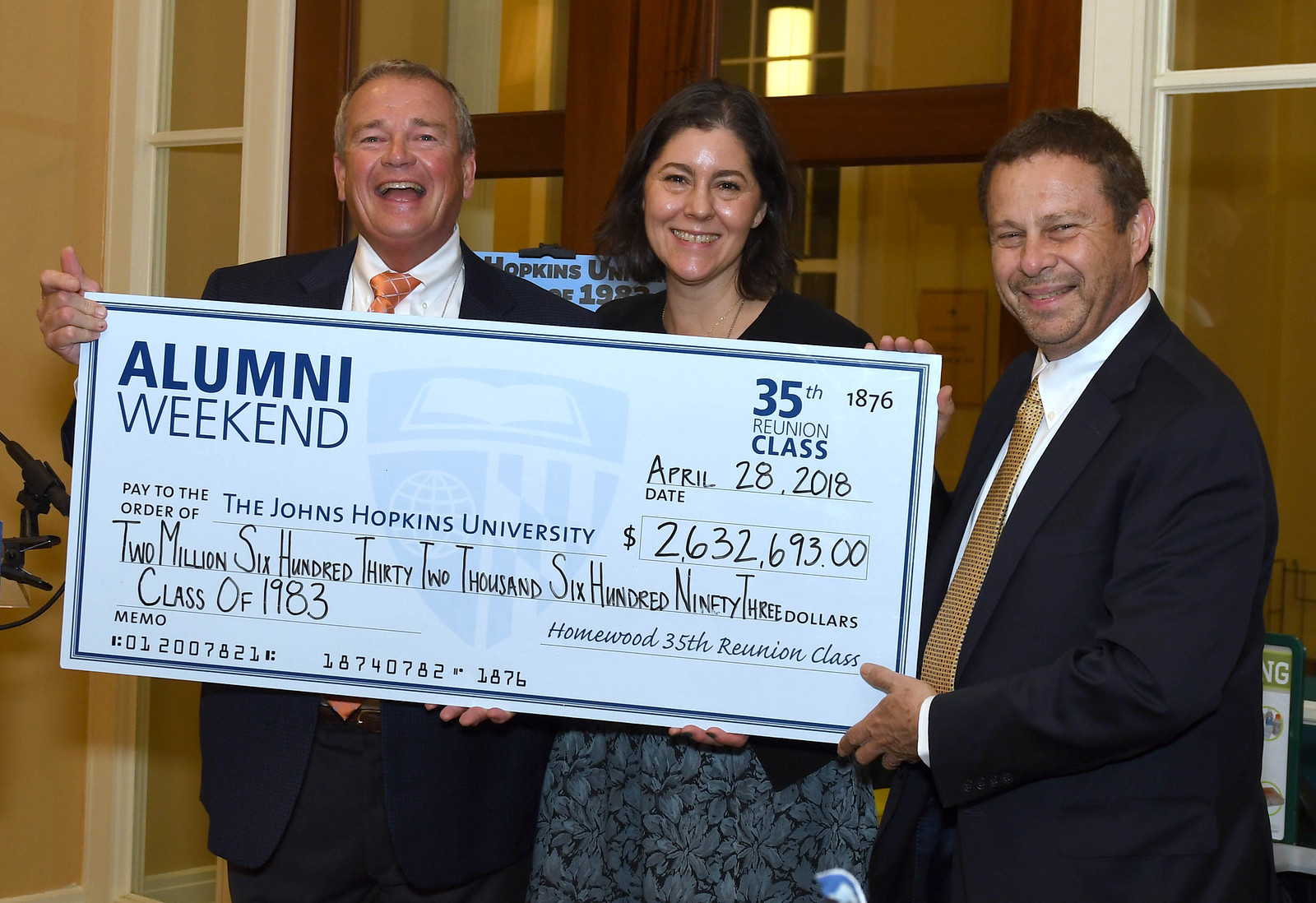In this indoor photograph, three people are standing side by side, posed in front of a window or doorway. On either side are two men in blue suits: the man on the left appears to be older and sports an orange tie, while the man on the right has curly brown hair and wears a gold tie. Centered between them is a woman with shoulder-length dark hair, dressed in a black top with a floral skirt. They are all smiling and looking at the camera as they hold up a giant check. The check prominently reads "Alumni Weekend," "35th Reunion Class," and "April 20th, 2018" at the top. It is made out to "Johns Hopkins University" for the amount of $2,632,693, donated by the Class of 1983 during their Homewood 35th reunion. The specific amount, "$2,632,693," is also written underneath.